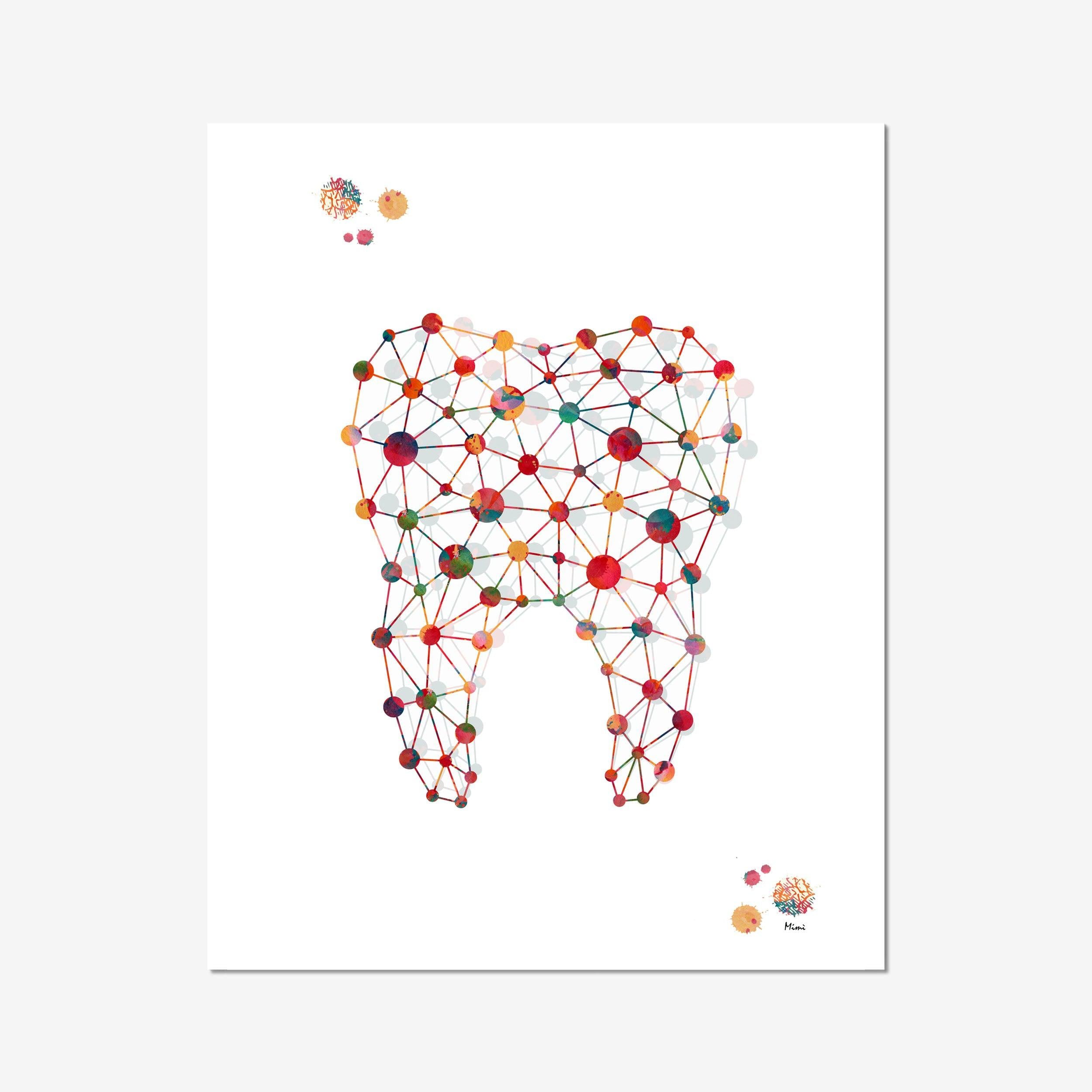This illustration depicts a tooth rendered in a cubism style on a white background, where the complex geometry of the tooth is built from numerous multicolored, marbled dots interconnected by lines. The dots vary in size and color, ranging from red and green to yellow and numerous mixes, giving the composition a dynamic and intricate appearance. The entire structure is outlined by a subtle drop shadow that adds depth and a three-dimensional effect to the design. Additionally, in the upper left and right corners, there are markings, likely the artist's signature or logo, accompanying a circle of multicolored dots and some text that is difficult to decipher. The bottom and right edges of the artwork feature a black line that may indicate part of the frame.